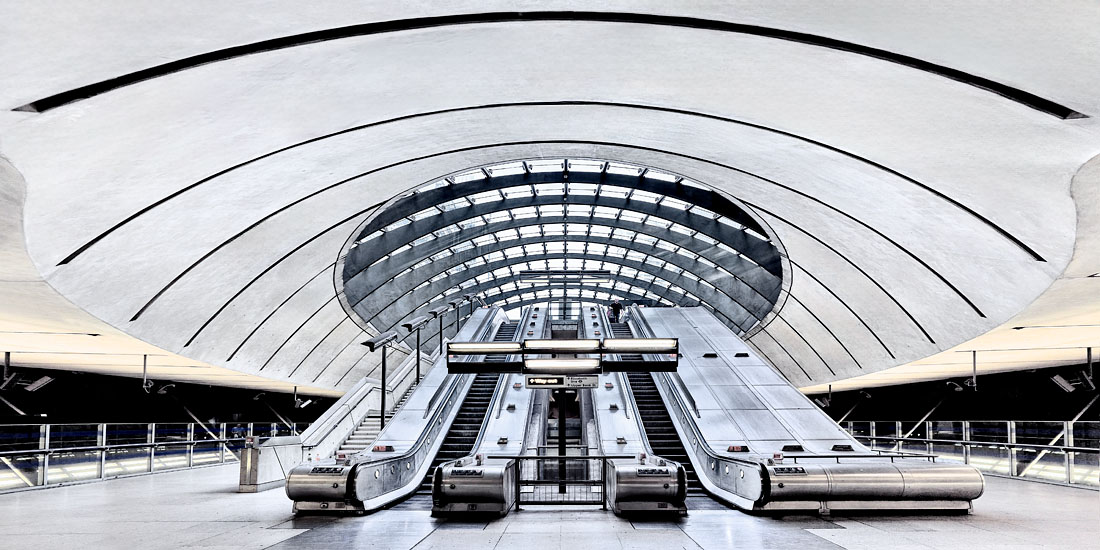This image captures a strikingly stark and spacious interior area dominated by polished silver escalators that ascend towards a grand, dome-like ceiling. The expansive room, devoid of people, creates a sense of vast emptiness and is characterized by its monochromatic color scheme of silver and gray, with minimal additional hues. Alongside the escalators, prominent railings or guardrails line the broad hallway, accentuating the space’s orderly design. Sparse black objects, potentially security cameras, can be spotted, hinting at a monitored environment. A sign with unreadable text is centrally positioned, adding to the mystery of the location, which resembles the sophisticated architecture often found in airports or large public lobbies. Overall, the image is a study in modern, utilitarian design, evoking curiosity about its purpose and use.